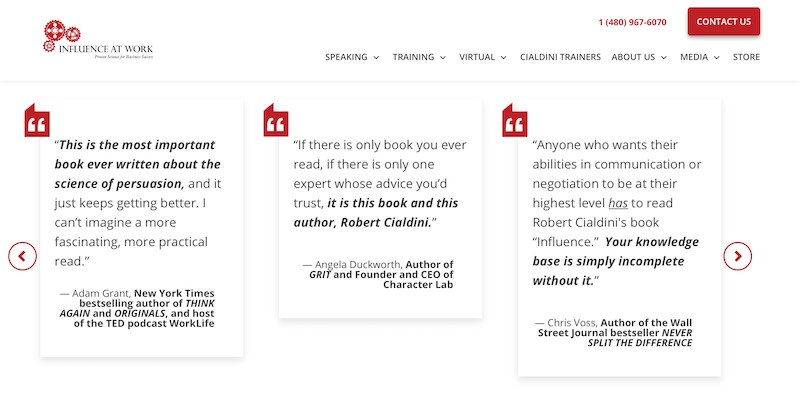In this image, we see the homepage of a website dedicated to the book "Influence at Work" by Robert Cialdini. The website's design is clean and professional, emphasizing the importance and impact of the book on the science of persuasion. 

In the top right corner, there is a contact phone number, 1480-967-6070, for visitors who wish to get in touch. Adjacent to the phone number, a conspicuous red "Contact Us" button likely provides further contact details and options.

Below the contact information, a navigation menu features several clickable sections in small gray text, including: Speaking, Training, Virtual, Calendar, Trainers, About Us, Media, and Store. Each section is designed to guide visitors through the various resources and services offered by the site.

The main content area displays three highlighted quotes from notable individuals, each enclosed within its own square. The first quote, located on the left, praises the book as "the most important book ever written about the science of persuasion," emphasizing its continuous improvement and practical value. 

The middle quote underscores the credibility and authority of the book, stating, "If there is only one book you ever read, it should be this book by Robert Cialdini," and attributes Cialdini as the founder of CEO Labs and Character Lab. 

The third quote, on the right, appeals to those seeking to enhance their communication and negotiation skills, insisting that "Influence" is a must-read for achieving the highest level of proficiency in these areas. 

From the content and layout, it is clear that the website serves to promote the book "Influence" by Robert Cialdini, offering information on speaking engagements, training programs, and additional resources for those interested in harnessing the power of influence and persuasion in their professional lives.